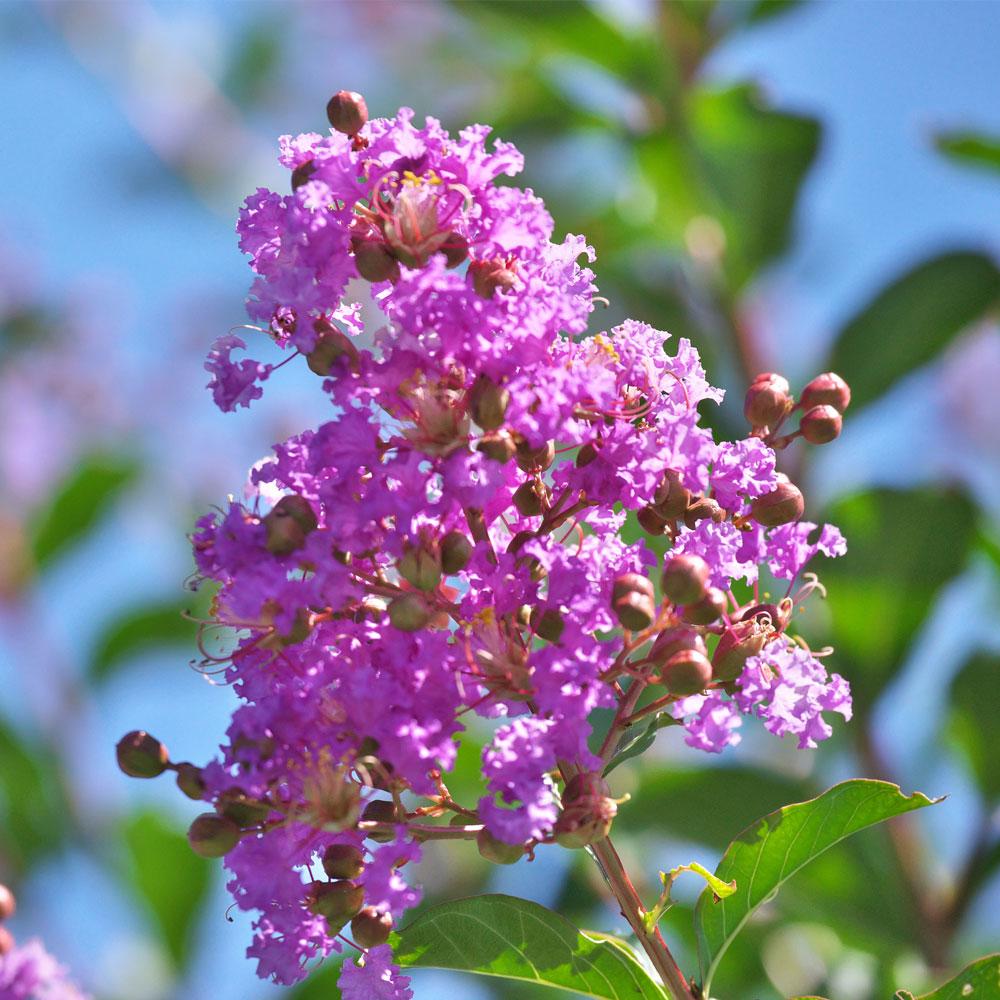This vividly detailed square photograph, approximately 6x6 inches, captures the outdoor beauty of a flowering plant in bright, natural daylight. The central focus of the image is a long, slender stalk that emerges just right of center from the bottom and extends almost to the top, leaning slightly towards the left. The stalk features vertical stripes of light tan and thin red hues. Surrounding the base are long, elliptical green leaves folded inward.

At the top of the stalk, the plant showcases an array of delicate pinkish-purple flower buds interspersed with small, hard, greenish berries just beginning to form. The flower petals, appearing puffed and ball-like, offer a textural contrast to the slender stalk.

The vibrant, sunny colors — purples, pinks, greens, and hints of yellow — are accentuated by the beautifully blurred backdrop of blue sky and additional green foliage. This sharp, close-up image immerses viewers in the wilderness, highlighting the intricate details and natural beauty of the plant.